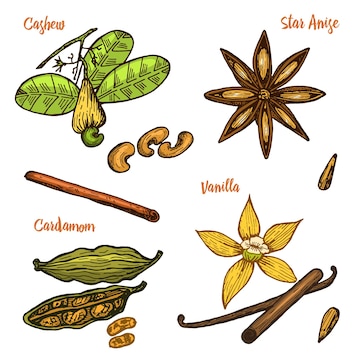The illustration presents a detailed depiction of various herbs and spices, each meticulously labeled except for one item. At the top left, the drawing showcases the cashew plant, featuring green leaves and a vibrant cashew fruit reminiscent of a fig with a small green nut attached at the bottom, alongside three roasted cashew nuts. Adjacent to it, on the top right, is the star anise, characterized by its distinctive eight-pointed star shape with tiny seeds nestled inside each segment. On the bottom left, the cardamom pod is illustrated, highlighting its green, cocoon-like appearance with numerous seeds inside, some of which are shown separated from the pod. Above the cardamom, though unlabeled, is a cinnamon stick, distinguishable by its curled bark appearance. To the right of the cinnamon is a vanilla flower, featuring five yellow petals with a white interior, accompanied by a depiction of the long, slender black vanilla bean with rounded tips.